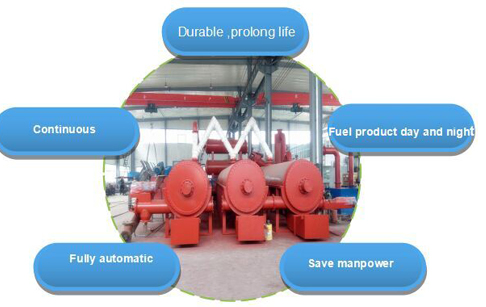This image, apparently designed for a website, features a simple graphic design with a central circular photograph, likely cropped, depicting a scene from a factory. The photograph shows industrial machinery, including three red cylindrical tanks with visible valves and pipes, set against a backdrop of a metal roof and concrete floor. The machinery is possibly some industrial hardware with red rails and white overhead pipes and an 'M' lettering on a part of it.

Surrounding the central image are five light blue oval bubbles with a subtle gradient color, darker at the bottom and lighter at the top, reminiscent of buttons from an old operating system. Each bubble contains white text detailing specific features or benefits, arranged clockwise like positions on a clock. At the top 12 o'clock position, the bubble reads "Durable, Prolonged Life". At 3 o'clock, the text "Fuel Product, Day and Night" is shown in a slightly bolder font. The 5 o'clock bubble states "Save Manpower". The 7 o'clock bubble is slightly off-center and reads "Fully Automatic". Lastly, at 9 o'clock, the bubble simply says "Continuous".

The meticulous arrangement and detailed descriptions within the bubbles suggest this image is intended to convey product features or benefits, likely showcasing advanced industrial machinery for a commercial purpose.